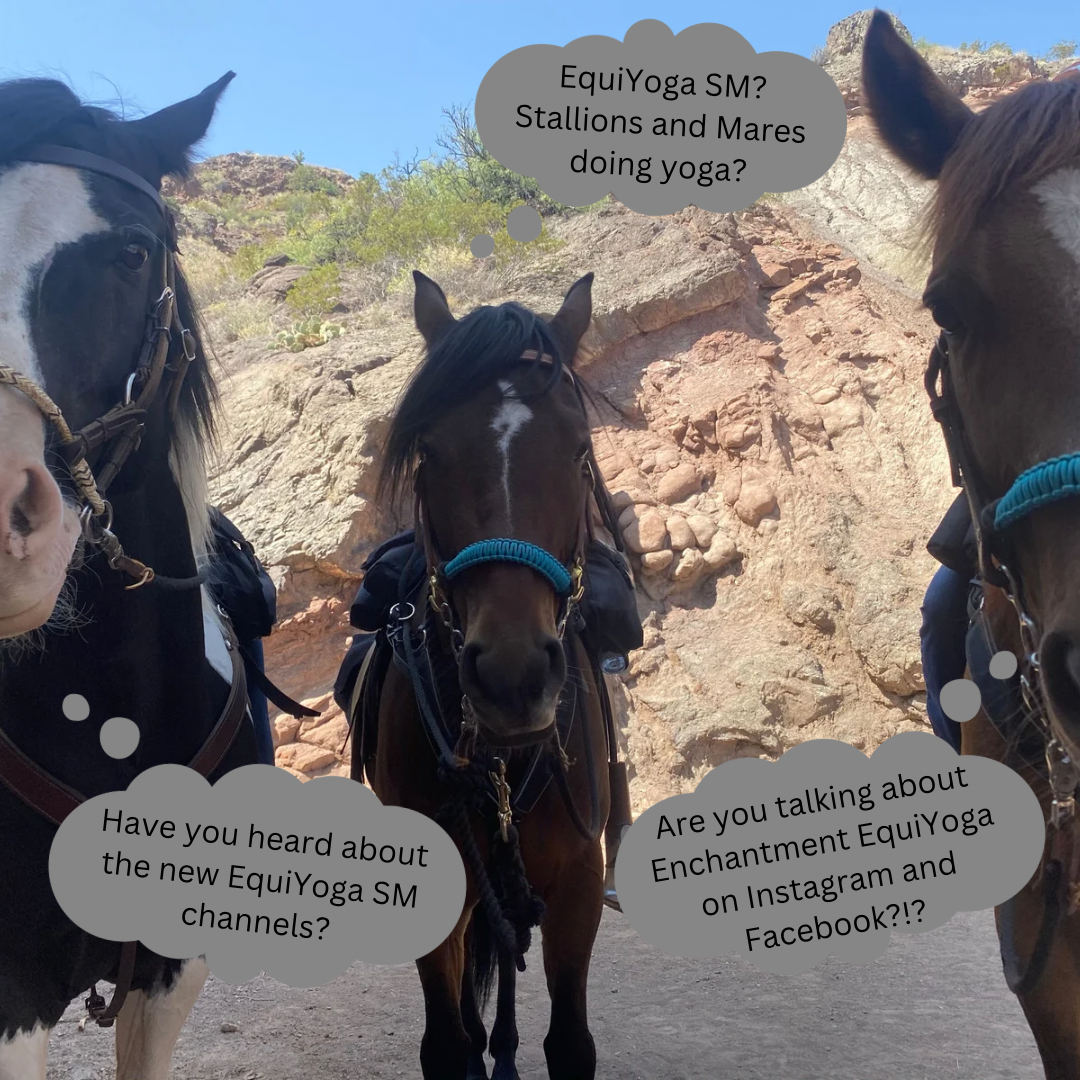In this striking image, three horses stand at eye level, closely staring into the camera, seemingly engaging with the viewer. They are situated in a canyon-like setting, with red clay rock formations surrounding them, casting gentle shadows over their figures. Each horse is fully saddled and bridled, equipped with saddle bags, but with no riders. Two of the horses are a rich brown with distinctive white stripes down their faces, while the third horse is black, also featuring a prominent white stripe. Notably, their bridles are color-coordinated— one horse wears a beige bridle, whereas the other two sport teal ones wrapped around their snouts.

Adding an unusual twist to this serene equestrian scene, three speech bubbles hover above the horses' heads, each like they're talking about "EquiYoga SM". They mention various things like "Have you heard about the new EquiYoga SM channels?", "Are you talking about Enchantment EquiYoga on Instagram and Facebook?", and "EquiYoga SM, stallions and mares doing yoga." These captions suggest that this image doubles as an advertisement for a yoga or wellness program, cleverly infusing an element of social media engagement.